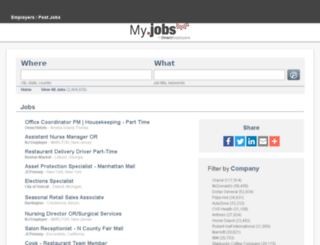This is a screenshot of the website MyJobs, which serves as a job board platform. The interface features a black header bar at the top, followed by a white navigation bar with the "MyJobs" logo prominently displayed. Below this, there is a gray search box that prompts users to enter keywords for job titles ("what") and locations ("where"). Beneath the search box is a list of job postings, although the text is too small to read clearly. The only legible job title includes the term "office."

On the right side of the page, there is a sharing option that allows users to share job postings on Facebook, Twitter, LinkedIn, via email, and by using a plus sign to add other sharing methods. Below the sharing options, there is a "Filter by Company" section, featuring a list of companies from which users can choose to filter job postings. Unfortunately, further details are difficult to discern due to the small font size, and attempts to enlarge the image only increase the size of the instructions, not the content. Overall, the image portrays the layout and some features of the job board, albeit with limited legibility of specific job listings.